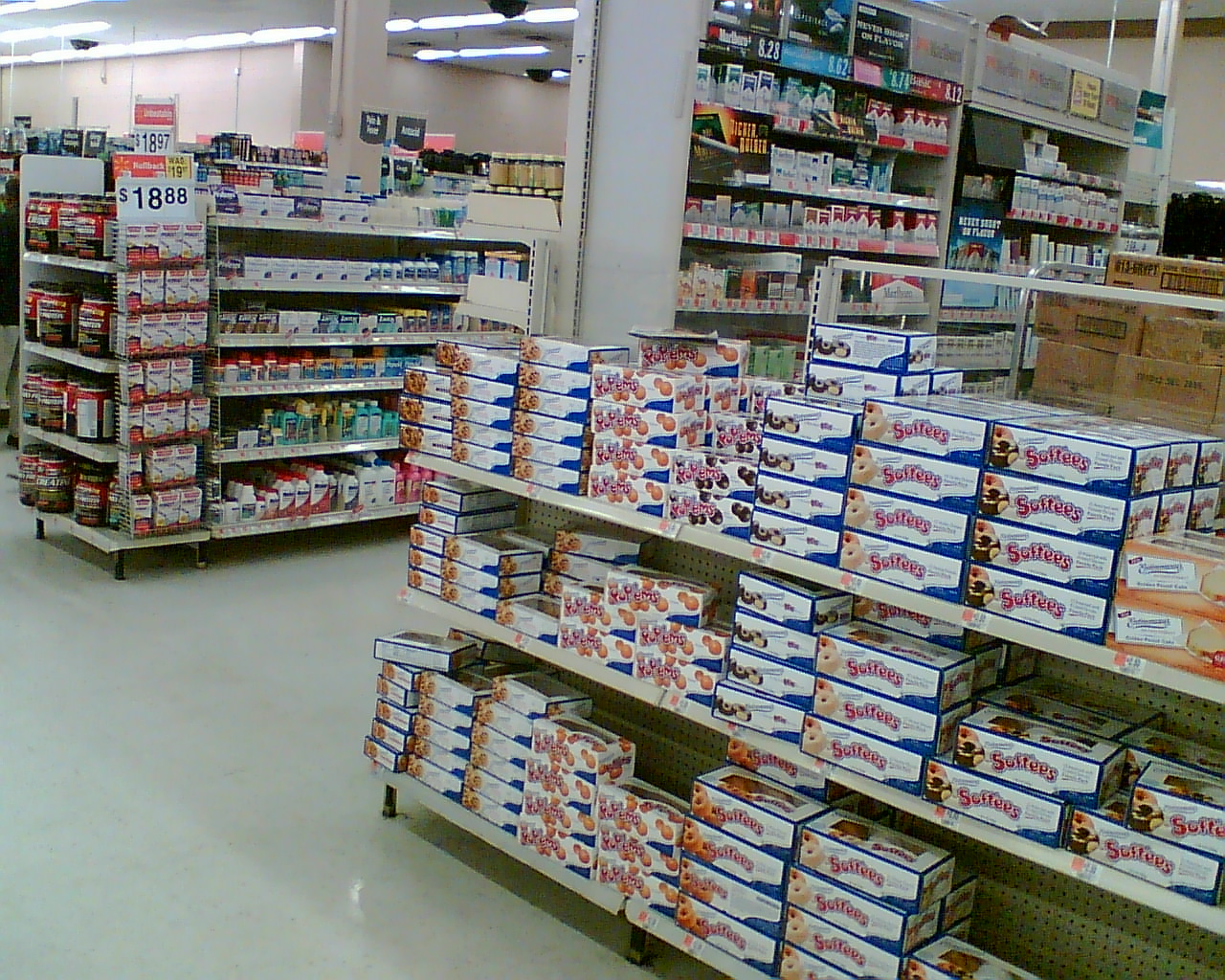In this image, we see the interior of a store, likely a market or pharmacy, featuring multiple aisles lined with various products. Dominating the foreground is an aisle with a prominent display of donuts, specifically boxed products from Sophie's Donuts. Adjacent to this, on the right-hand side of the image, there are packages of Entenmann's snacks, recognizable by their branding.

In the background, another aisle appears to be stocked with cigarette packs. To the left side of the image, a price tag indicates an item costing $18.88, though the specific product is indiscernible. This section of the aisle might be dedicated to medicines, as it includes blue bottles, possibly of Vinelanta, among other medicinal products and perhaps whey protein containers.

Additionally, the image is illuminated by fluorescent lights mounted on the ceiling, casting a uniform glow across the rows of assorted items whose specific identities remain unclear. The overall scene captures the bustling, organized environment typical of a retail store.